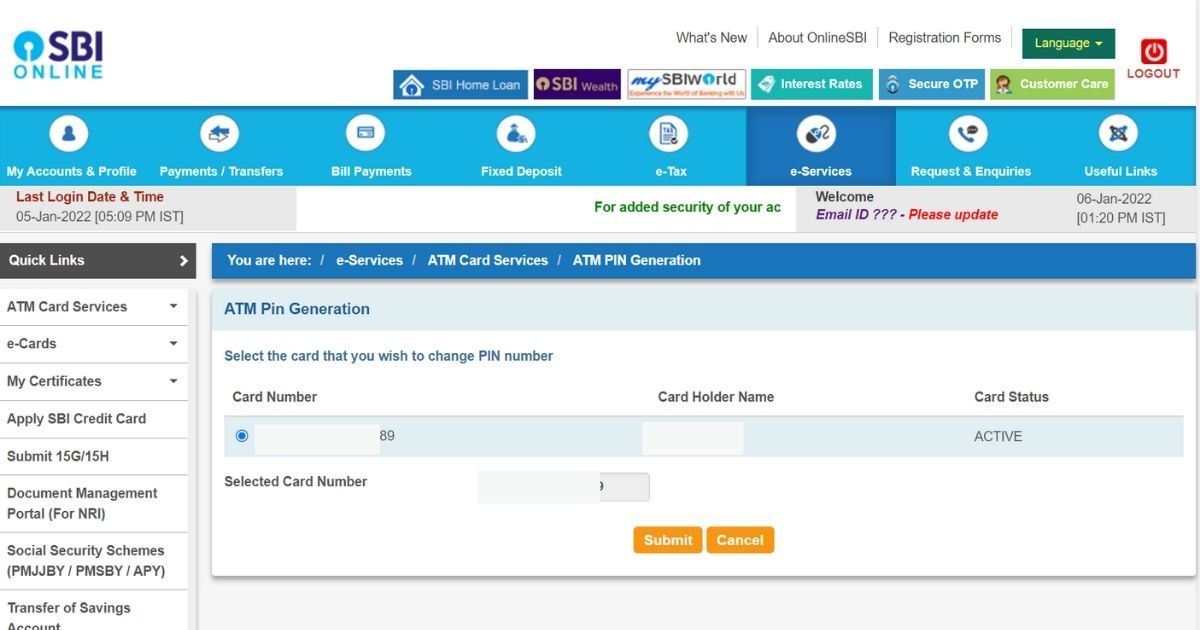The image depicts a detailed web interface for SBI Online. In the upper left corner, there is the SBI Online logo, which features the letters "SBI" in dark navy blue positioned above the word "Online" in aqua blue. Adjacent to the text, there is a small aqua icon that resembles a turntable record or a fan, contributing to the logo's design.

To the right of the logo, there are several clickable buttons aligned horizontally on a medium aqua border that separates the top section from the rest of the page. From left to right, these buttons include:
   1. **SBI Home Loan** (with an icon on a medium pale blue background)
   2. **SBI Wealth** (on a background transitioning from navy blue to almost purple)
   3. **My SBI World** (against a white background, promoting the experience of global banking with SBI)
   4. **Interest Rates**
   5. **Secure OTP**
   6. **Customer Care**
   7. **Log Out**

Below the aqua border, there is a horizontal menu with white text on the aqua background, listing navigation options such as:
   - My Accounts and Profile
   - Payments/Transfers
   - Bill Payments
   - Fixed Deposit
   - E-Tax
   - E-Services
   - Requests and Inquiries
   - Useful Links

Additionally, there is information about the last login date and time displayed to the left, under the blue banner.

On the left side of the main section, there is a vertical column containing various links and subsections in a secondary menu. These include:
   - Quick Links (currently selected)
   - ATM Card Services
   - E-Cards
   - My Certificates
   - Apply SBI Credit Card
   - Submit Form 15G (and other forms or related services)

Occupying the central section of the webpage, under the horizontal blue banner, is a 'You are here' navigation indicator for "E-Services > ATM Card Services > ATM Pin Generation". This section features a form titled "ATM Pin Generation", instructing the user to select the card they wish to change the PIN for. The form includes blank fields for Card Number, Cardholder Name, and Card Status, with options to Submit or Cancel the changes.

The overall design includes a mix of blue tones and white, emphasizing a clean and professional layout typical for banking websites.